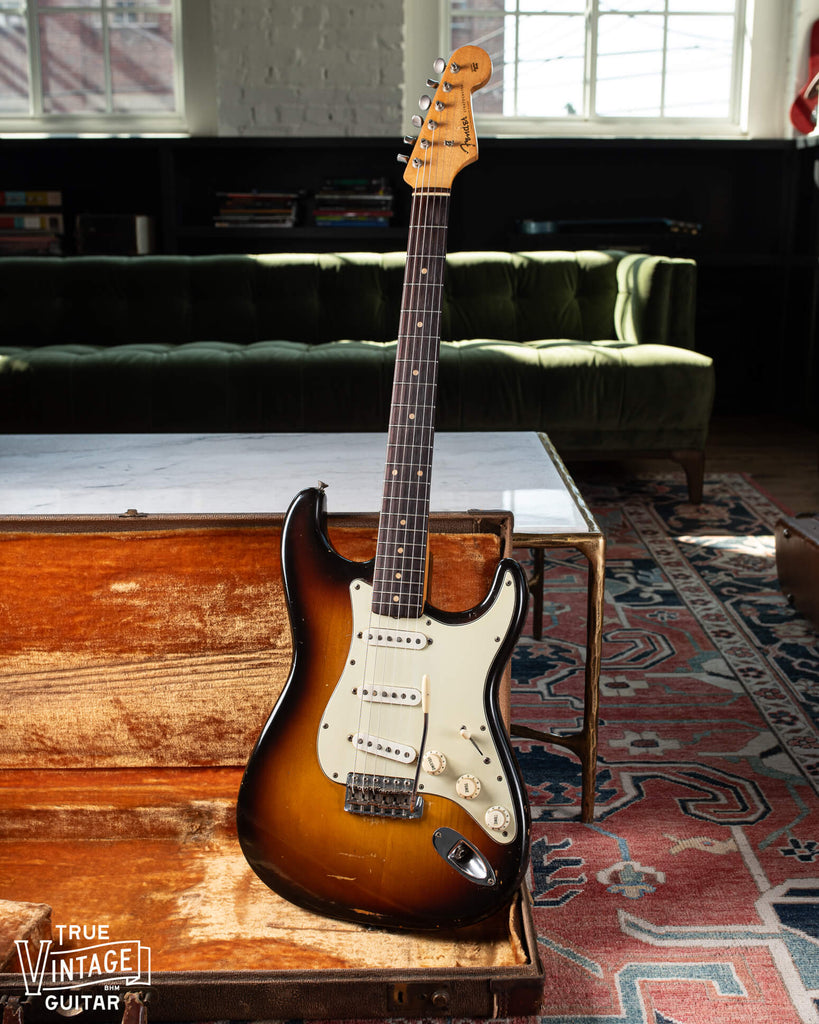The image depicts a shiny electric guitar prominently positioned upright in the middle of a living room. The guitar has a striking mix of brown, white, and black with a black fretboard. It stands in a wooden case placed on a large, red geometric-patterned rug that covers much of the living room floor. Behind the guitar, a green sofa is bathed in sunlight streaming through open windows, which are white-framed and allowing light to spill onto the sofa, table, and rug. The guitar, which appears well-tuned, is clearly a Fender, showcasing detailed tuning pegs on its long neck. In the bottom left corner of the image, “True Vintage Guitar” is inscribed in white text, emphasizing the musical and vintage theme of the scene.